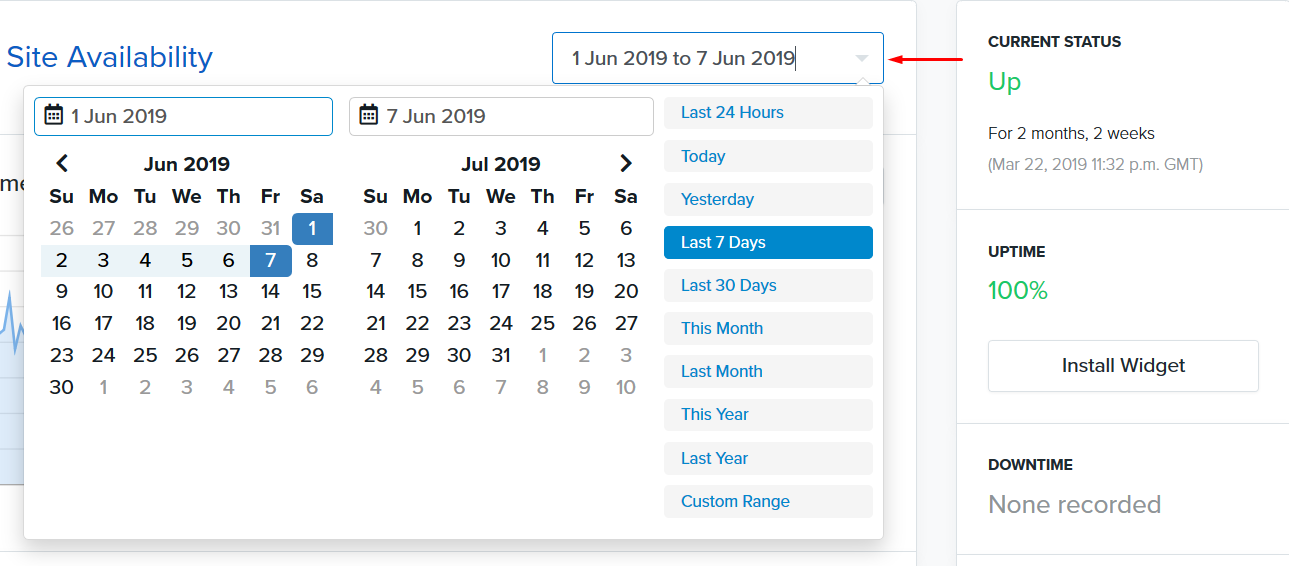The image depicts a calendar interface showing site availability from June 1, 2019, to June 7, 2019. The selected date range is displayed in a drop-down menu located at the top right corner of the calendar, with the text "1 Jun 2019 to 7 Jun 2019" without an 'e' in June. The highlighted dates, June 1 to June 7, are marked in blue, while the remaining dates appear in white against a black background.

To the right of the calendar, there's a blue button labeled "Last 7 Days," accompanied by a list of other date range options, including "Last 24 Hours," "Today," "Yesterday," "Last 30 Days," "This Month," "Last Month," "This Year," "Last Year," and "Custom Range." Adjacent to this list is an arrow pointing towards the drop-down button, and to the right of the arrow, green text indicates the "Current Status," showing the site has been up for 2 months and 2 weeks with a 100% uptime.

Below this status indicator, there's a button for installing a widget. Additionally, the section below indicates "Downtime" in black, with "None Recorded" written in light gray. Hidden beneath the calendar pop-ups, on the middle left side of the image, is a graph depicting site availability, set against an all-white background, which includes a condensed view of June 2019 and July 2019.